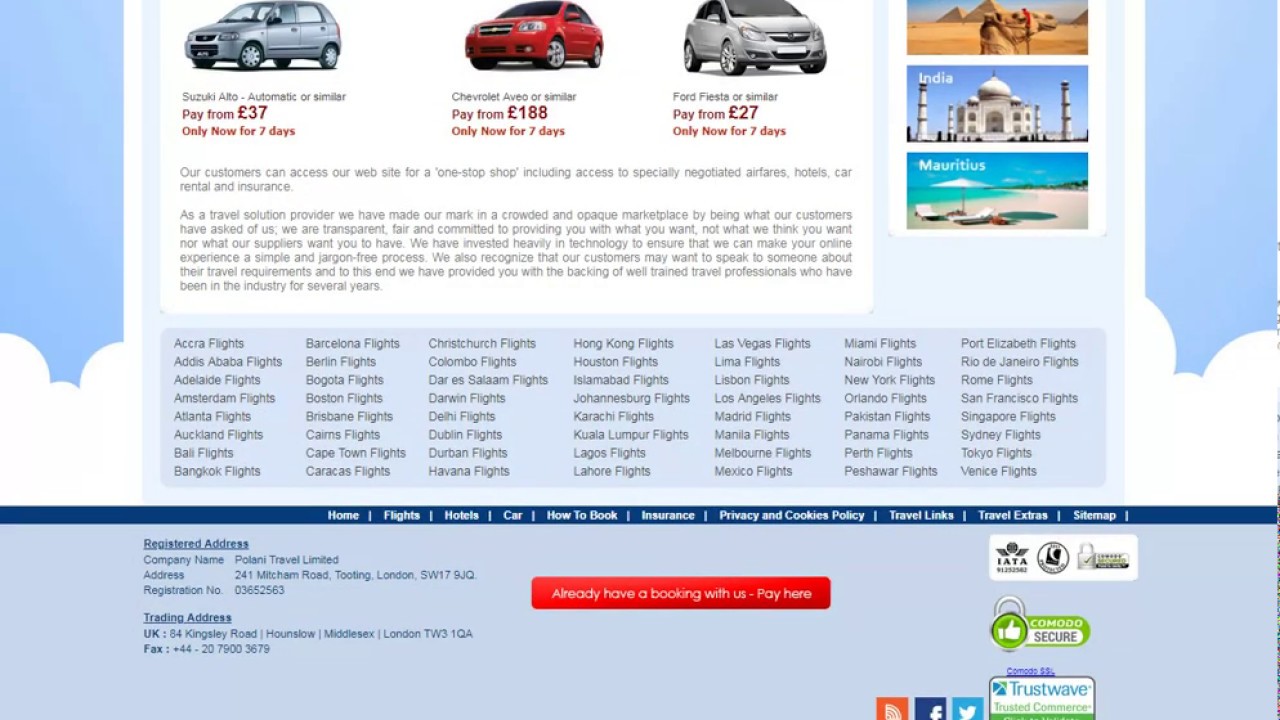**Detailed Screenshot Description:**

The screenshot captures the bottom section of a travel-related website. The upper part of the screenshot features images of three rental cars prominently displayed with their respective rental rates. On the left, there is a Suzuki available from £37, in the center is a Chevy Aveo available from £188, and on the right is a Ford Fiesta, available from £27. 

Beneath the car listings, there is a paragraph of text, although the content is somewhat difficult to read in detail. The text appears to pertain to the travel services offered by the website, likely providing information or promotional content.

Below this paragraph, there is an extensive list of text links categorized under various city names, presumably for search engine optimization (SEO) purposes. These links suggest flight destinations and are structured into 7 columns, with 8 flight destinations listed in each column. Some of the cities mentioned include Accra and Addis Ababa, among others.